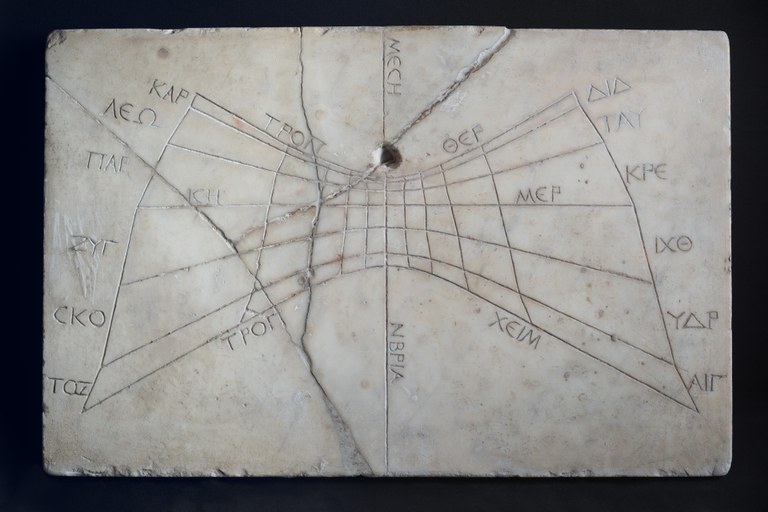The image is a detailed photograph of an engraved piece of white marble, showcasing a complex, three-dimensional plane or geometric shape that resembles a bow tie. This plane warps in the middle and spreads out toward the edges, creating a sense of depth and perspective. The surface of the marble is very smooth, intersected by a grid of horizontal and vertical lines, creating a checker pattern. The left side of the marble features notable cracks, and there is a small hole slightly below the top center that resembles a bullet hole. Along the edges of the engraved plane, there are numerous Greek letters labeling various parts of the grid, including the center line, top and bottom edges, and lateral lines. The photograph is set against a black backdrop, emphasizing the intricate details and textures of the marble engraving.